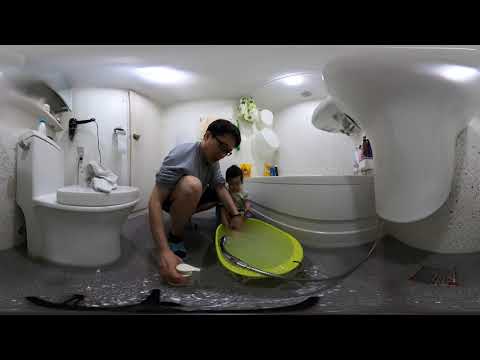In this detailed image, a man of Asian descent, approximately 30 years old with short black hair and glasses, is seen in a white bathroom with his young child, possibly a toddler. The father is squatting beside a green bathtub, filling it with water using a shower head. He also holds a bottle of lotion in his other hand. The room features white walls, a white ceiling with several ceiling lights, and a floor that appears wet. To the left of the man, there's a closed white toilet with a crumpled towel on top, and next to it is a hair blow dryer. On the right side, the bathtub is visible alongside the bottom part of a sink. Soap and shampoo are available for use. The photo, likely taken with a fisheye lens, also shows a bathroom door and gives a wide view of the space, suggesting a bustling bath-time preparation.